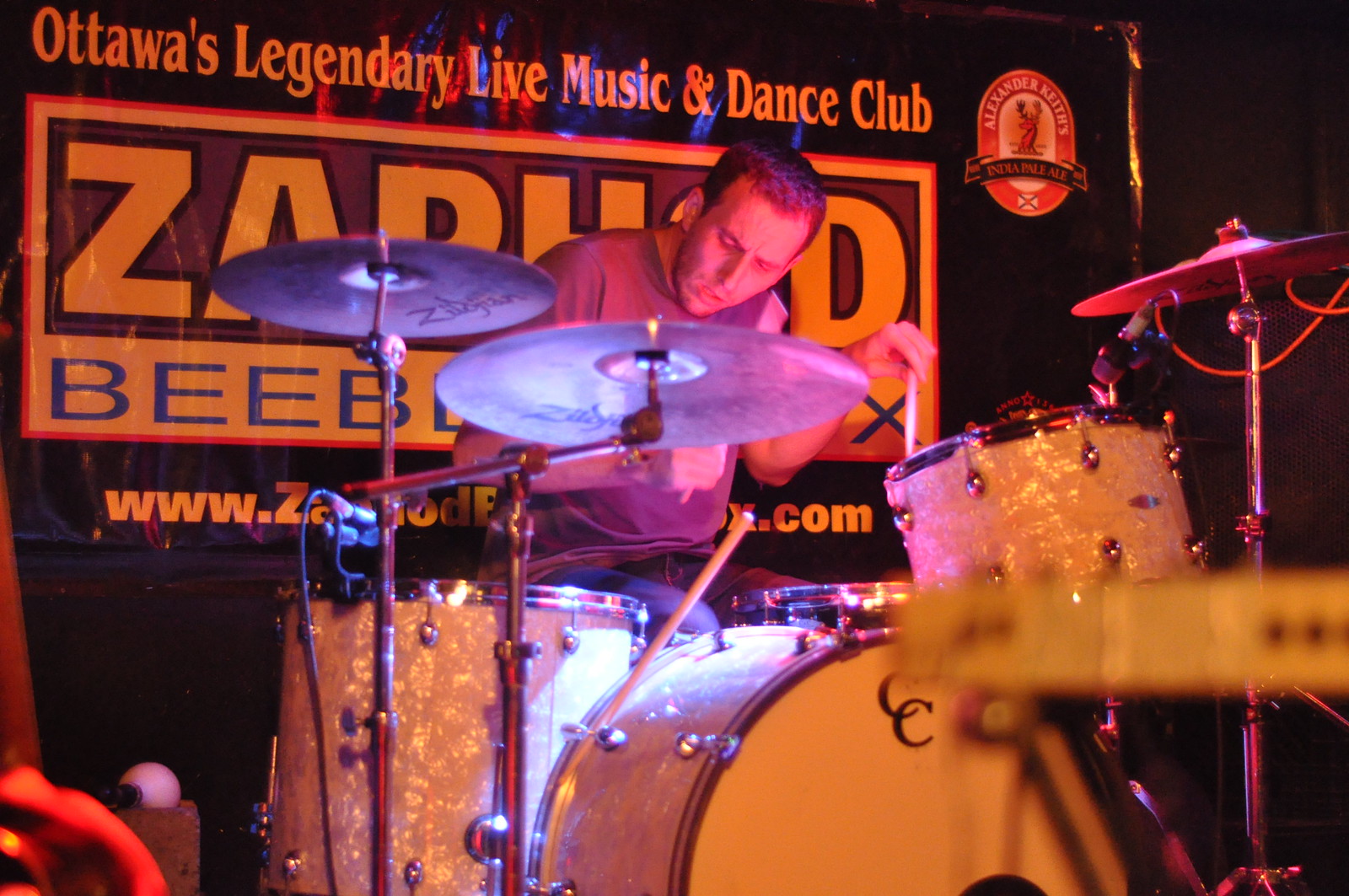This color photograph captures a drummer immersed in his performance, bathed in a pinkish-red light that lends a warm glow to the scene. He is seated behind an elaborate drum kit, which features white sparkles on the drums and a bass drum prominently displaying the letters 'CC'. The man is wearing a gray shirt, although the reflections make it appear reddish, with his head tilted down and to the right, concentrating on his craft. He holds drumsticks in his hands, poised above two cymbals positioned in front of him, and additional cymbals and drums complete the set.

Behind the drummer is a vibrant sign with yellow text on a black background. The sign reads "Ottawa's Legendary Live Music and Dance Club," but part of the banner, starting with the letter 'Z', is obscured by the man and his drum kit. Below this text, there appears to be a web address; however, only portions of it are visible, showing 'www.Z' at the beginning and '.com' at the end. To the right of the man, level with his shoulders, stands another cymbal. The backdrop behind the drummer is entirely black, accentuating his illuminated figure and the detailed intricacies of his drum kit.